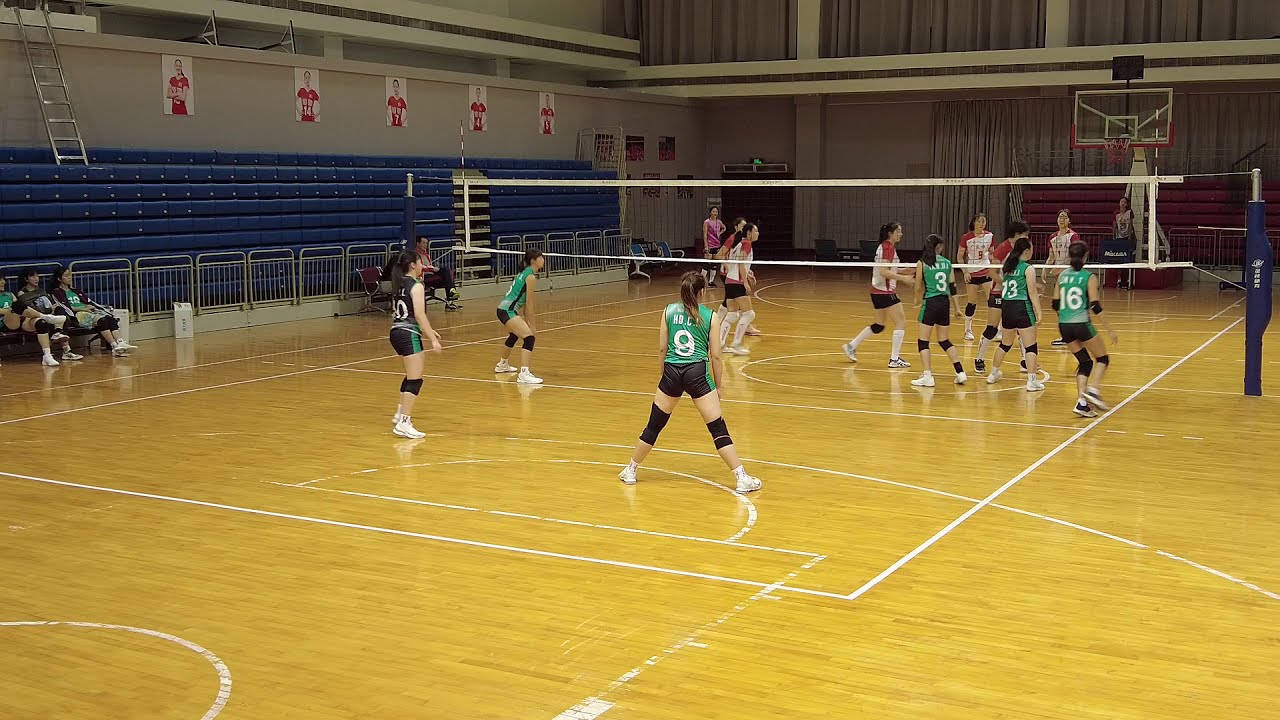The image depicts a high school girls' volleyball game set in an indoor gymnasium that doubles as a basketball court. The gym's wooden floor is marked by a white volleyball net set at girls' height. In the foreground, the team closest to the camera is outfitted in green jerseys with black shorts, and their libero is distinguishable by her black jersey. Opposing them on the other side of the net, the second team wears red and white jerseys with black shorts. Both teams' players are actively engaged in play, with three blockers positioned at the net on the right side. There might be a coach in the background, providing guidance. The gym features blue bleachers to the left, which are retracted and empty, though a few players sit on folding chairs before them. A basketball hoop is visible in the background, indicating the gym's dual purpose. The absent volleyball itself does not detract from the anticipation of the players, some of whom appear poised to react to its flight.